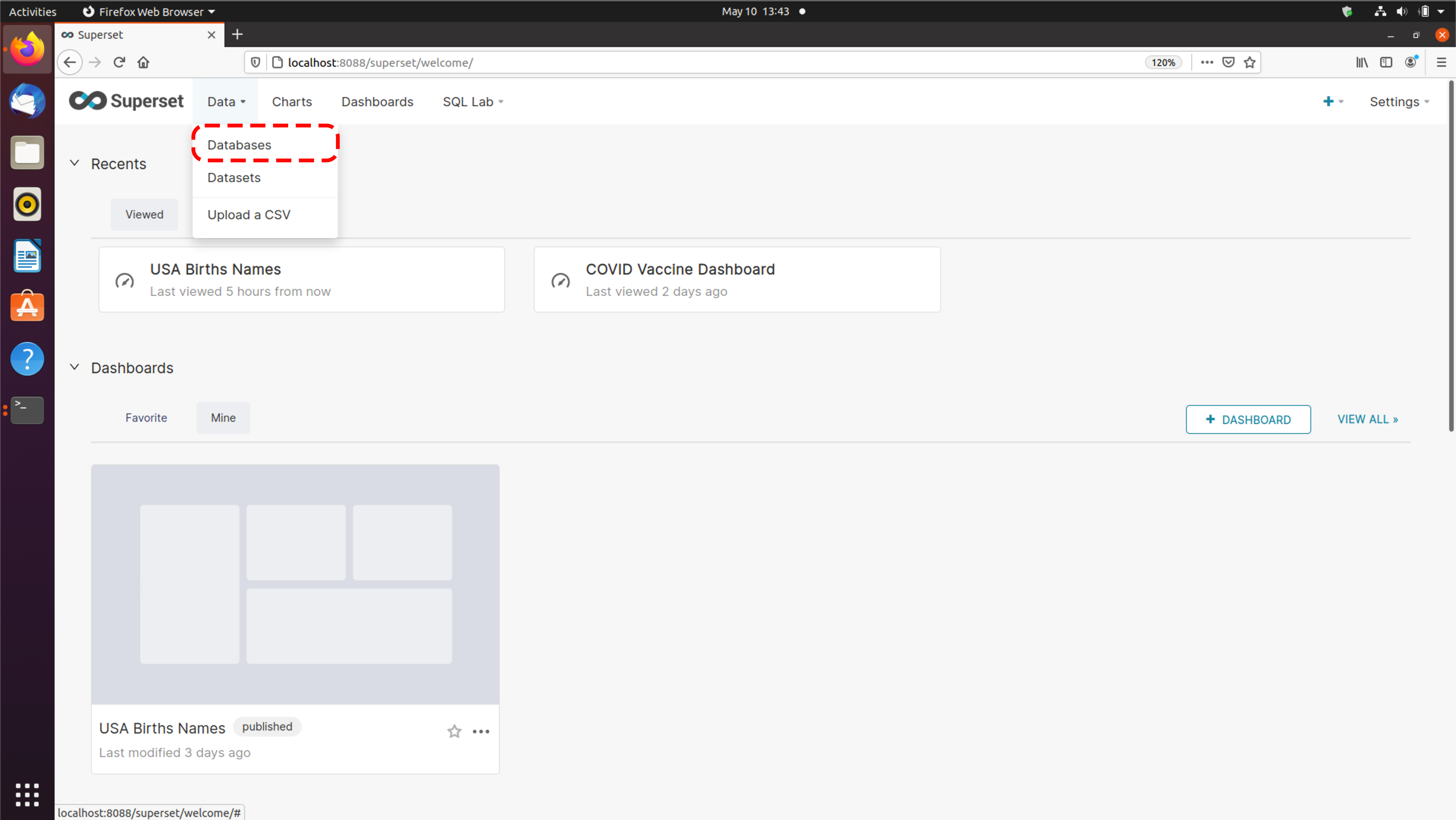The image displays a detailed view of a computer screen, showcasing a user interface loaded with various elements and data points. At the center of the screen is the date "May 13th, 1343" in white text, standing out against a primarily black background.

On the left side, vertically aligned, are several icons: the Firefox logo, a blue circle featuring a white envelope, a gray square containing a white envelope, a white square with an orange and black circle, and a white and blue sheet of paper. Further down are an orange suitcase with a white 'A' inside, a blue circle with a question mark, and a gray circle. At the very bottom, there is an arrangement of nine dots within a square.

To the upper right, the title "Superset" is displayed within a gray box outline. Nearby are a left arrow inside a white circle, a gray circle representing the refresh button, and some text. Below that, a blue number "8" is visible with "Superset" to the side, followed by sections labeled "data," "charts," "dashboard," "SQL lab," and "settings." Under the "data" section, specific listings include "databases" surrounded by red dots, "data sets," and "upload a CSV."

To the left, a drop-down menu labeled "recents" with an arrow down is present, above a gray box marked "viewed." Adjacent entries include "US birth names," last viewed five hours ago, and "COVID vaccine dashboard," last viewed two days ago. Further down, a section labeled “dashboards,” includes options for "favorite" and "more" within gray squares. Another section features a “dashboard” button against a white background with a blue square, next to a "view all" link.

At the bottom left, a gray square contains four smaller, lighter gray squares in a specific arrangement. Below it, on a white background, is the text "US birth names," marked as "published," accompanied by another gray square with a star and three dots beside it. Lastly, the phrase "last modified three days ago" is listed underneath.